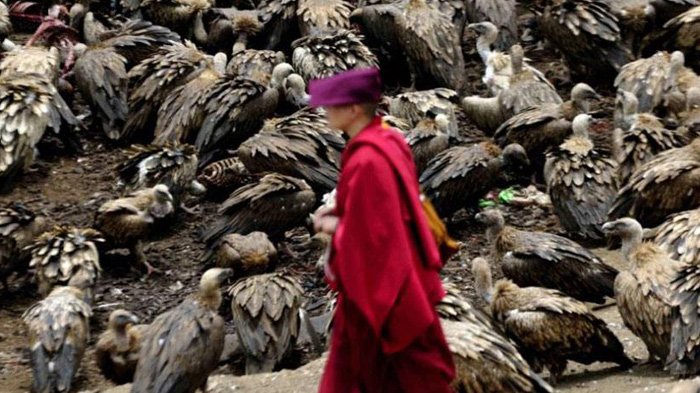This realistic photograph, taken by a photographer without the use of painting, drawing, or AI technology, captures an outdoor scene with a stark and desolate atmosphere. In the center stands a woman dressed in a long red robe, resembling a monk's attire, with a red cape or smock draped over her shoulders. She wears a distinctive purple hat that sits on the back of her head, extending forward like a bonnet. A brown satchel or backpack rests on her right shoulder as she walks, adding motion to the image. Surrounding her, the background teems with dozens upon dozens of large vultures, characterized by their dark to light brown feathers and gray heads. These vultures are scattered across a barren, dirt-filled landscape, some walking, most sitting, and seemingly engaged in milling about—potentially scavenging for food. The scene is devoid of text, allowing the vivid colors—red, yellow, purple, brown, black, white, teal, and dark orange—to enhance the visual impact of this intriguing and eerie tableau.